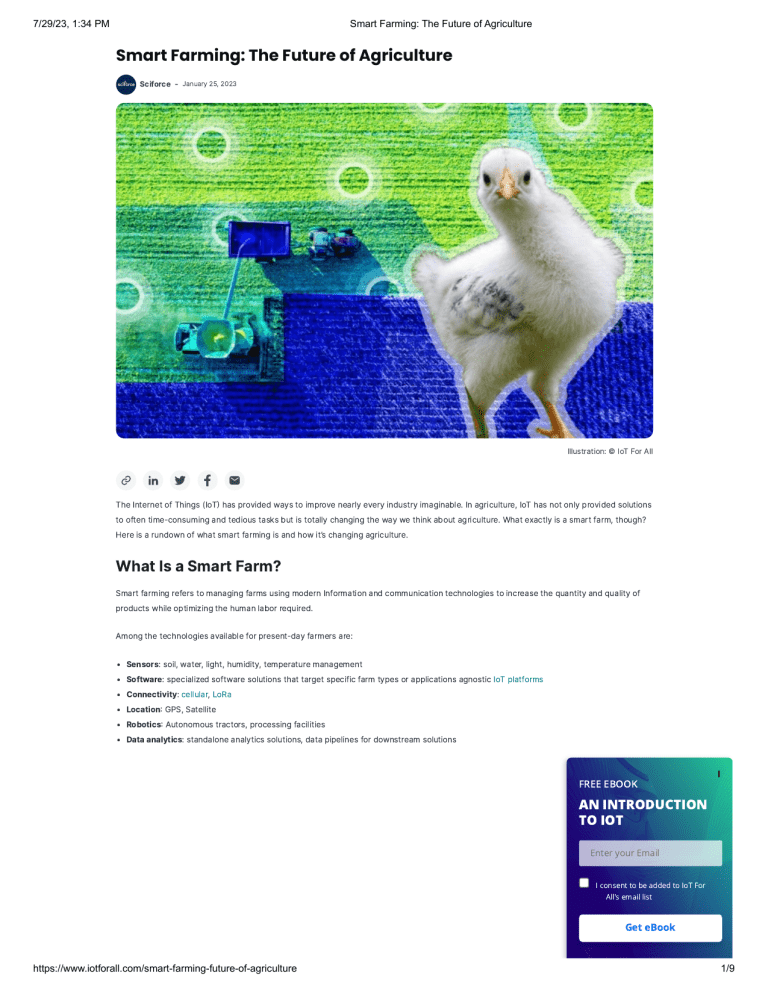On a webpage with a white background, the top left corner displays the timestamp "7-29-23-1:34 PM." Centered on the page, in bold lettering, it reads "Smart Farming, the Future of Agriculture." Beneath this, aligned with the "M" in "Farming," and continuing downwards, it is white again. Bolded in black text, it repeats "Smart Farming, the Future of Agriculture." Below this phrase is a small blue circle with illegible white text inside, and beside it, "Salesforce" is written along with the date June 25th, 2023.

Further down, there's an intriguing image as the focal point. The upper third of the picture is shaded in light green, transitioning into dark green in the middle, and finally dark blue at the bottom. Scattered around the picture are small white circles. Dominating the scene, a blue tractor with a blue trailer is positioned in the center. To its left, another teal tractor is visible. A prominent figure in the image is a small white chick situated in the right corner, standing upright with its chest facing left and gazing directly at the camera. The chick's beak and feet are orange, eyes black.

At the bottom right corner of this image is the word "Illustrations." Below the image, there are four social media links: Facebook, Twitter, LinkedIn, and an email link. 

Following the social media links is a section containing brief informational text spanning three lines. This is promptly followed by a bolded question: "What is a State Farm?" Two lines of white space precede another single line of content. 

Following this, there are six vertical dots paired with six bold-heading words or acronym signifiers arranged horizontally, each followed by a line of descriptive information.

In the bottom right corner of the webpage, there is a squared section divided into two halves: the left half in dark blue and the right in teal, with white text overlaying both sides. This section includes a search tab and a white button at the bottom reading, "Get a Book and Believe."